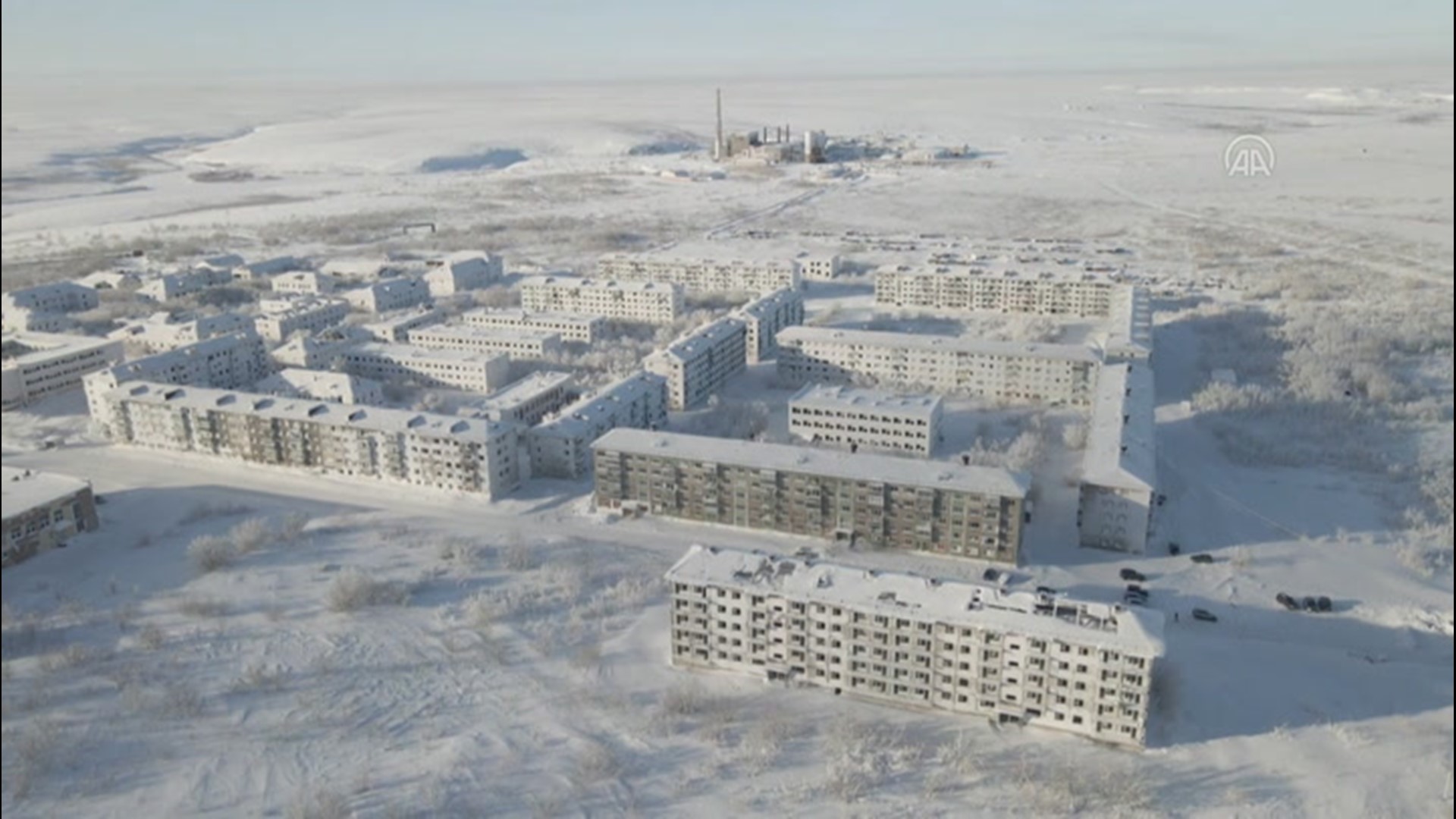This aerial color photograph captures a wintery scene of a small city, likely in the Arctic or Siberia. The entire landscape is blanketed in snow, giving everything a pristine white appearance accentuated by grayish hues. In the foreground, clusters of five-story apartment buildings with snow-covered roofs are arranged in organized squares around central courtyards, interspersed with snow-laden trees. To the lower left, a distinct large building stands separate from the apartments. At the horizon, a notable feature is an industrial facility, characterized by its prominent smokestack and large tanks, hinting at its function as a power plant. Beyond this facility, a vast frozen plain stretches out, possibly cradling a river, under a light blue and slightly greenish sky. The scene is sparse with vehicles, reinforcing the impression of a cold, snow-covered, tranquil urban area in the depths of winter.